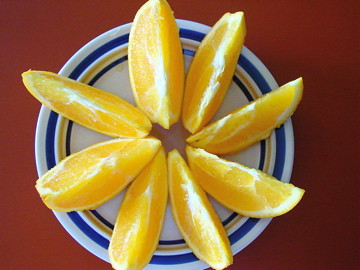In this detailed top-down photo, we see a white plate adorned with concentric rings of blue and yellow around its outer edge, resting on a red tabletop. Inside the plate, eight pale orange slices (possibly lemon given their light color and appearance) are meticulously arranged in a flower-like pattern. Each slice, roughly two inches long, reveals a small white pulpy center and a faint white rind on the outside. The image is closely-cropped, focusing solely on the plate and its decorative arrangement of fruit slices.